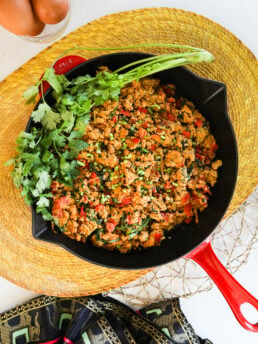This indoor photo, taken from a bird's eye view, showcases a culinary setup atop a light-colored, possibly white, table or counter. The central focus is a black cast iron skillet with a red handle, sitting on a woven placemat, potentially bamboo. The skillet contains a dish likely made of chicken and assorted vegetables, garnished generously with cilantro, adding both flavor and a vibrant green contrast. In the top left corner, there is a glass bowl containing brown eggs, enhancing the rustic and homely vibe of the scene. At the bottom, a colorful, folded cloth napkin in shades of blue, red, and gold adds a decorative touch. This composition, resembling those popular on culinary blogs or Pinterest, could be the work of a food influencer sharing a recipe.